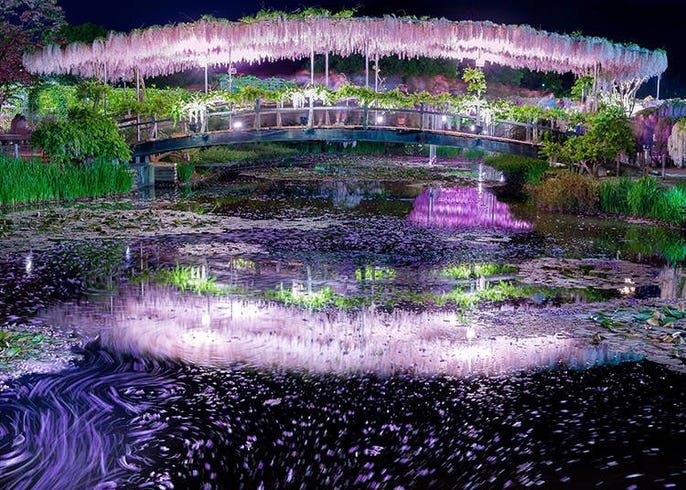The image depicts a phantasmagorical nighttime scene of a beautifully stylized bridge arcing over a tranquil river, framed by lush greenery. The bridge is adorned with a canopy featuring purple fringe that emits a soft, glowing light, creating an enchanting purple luminescence reflected in the water below. The railing of the bridge is lavishly decorated with vibrant foliage and delicate white flowers. In the water, purple flowers and floating leaves add to the magical atmosphere, while subtle streaks of purple hues scatter across the surface. Dominated by colors of pinks, purples, lavenders, and hints of green, the entire setting exudes a dreamlike quality. To the side, a walkway under a covering laced with hanging, cherry blossom-like strands and surrounded by large, ethereal trees enhances the fairy-tale ambiance. The scene is illuminated by an indirect light source that makes the flowers glisten, weaving together a vision of serene and surreal beauty.